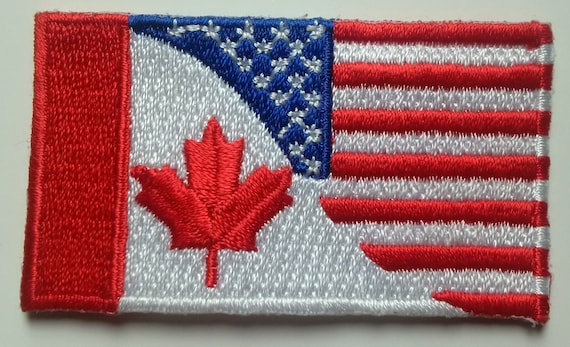The image depicts a rectangular embroidered patch made of intricate, woven fabric strands, designed to be sewn onto clothing like a shirt or jacket. This unique patch masterfully combines elements of the national flags of Canada and the USA. On the left-hand side, it features a red vertical rectangle characteristic of the Canadian flag, with a red maple leaf prominently displayed on a white background. A distinctive, curving line runs from the top left, meandering down into the center, and finally arches to the lower right, marking the boundary between the two flags. On the right-hand side, the patch displays the American flag's iconic design, complete with red and white stripes running vertically and a small section of blue containing silver stars. This visually striking patch symbolizes the blend of two national identities with a seamless, artistic flair.